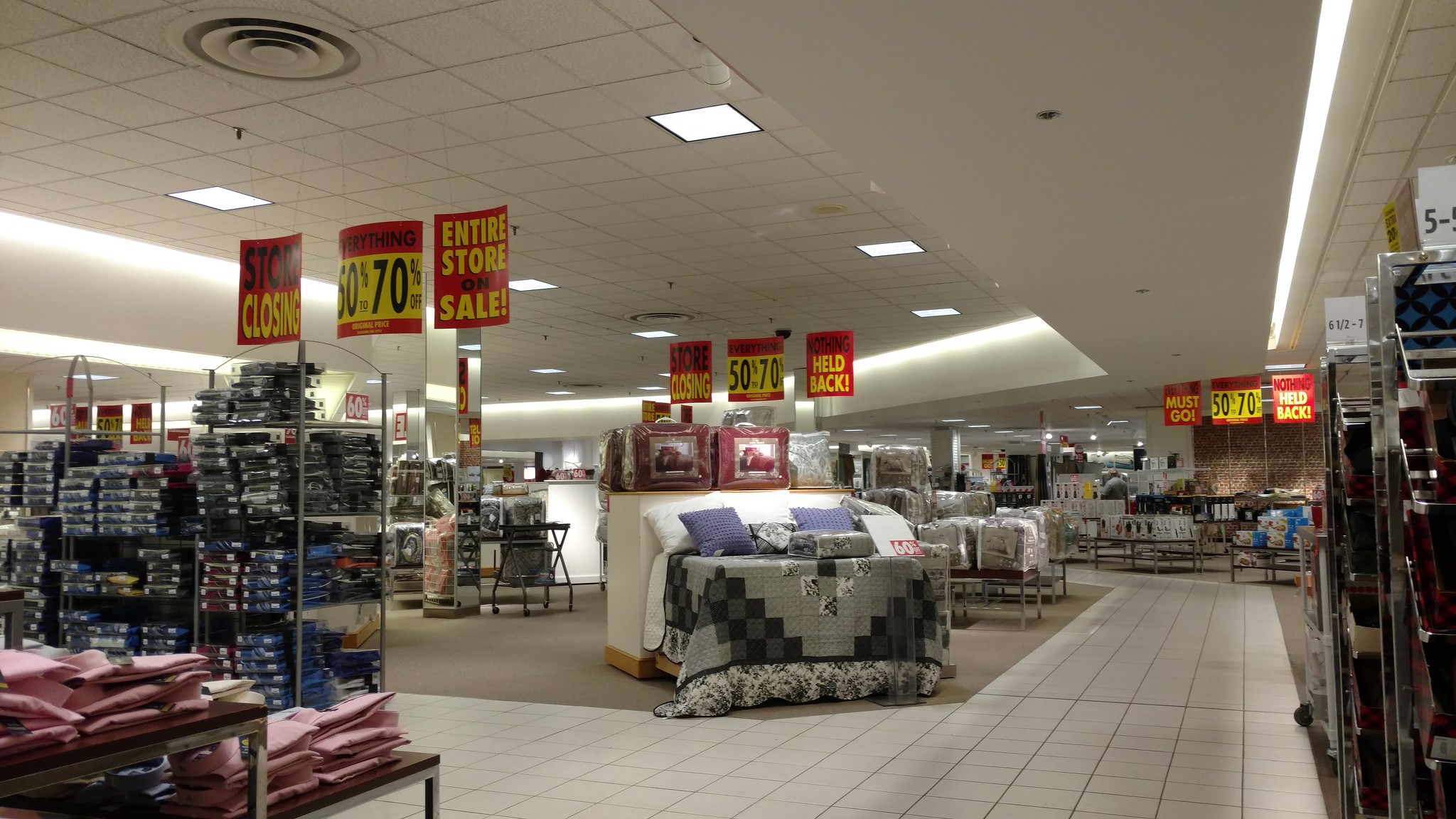This photograph captures the linen department of a department store in the midst of a closing sale. The scene features a combination of white tiled and tan carpeted flooring, with various display racks arranged throughout the area. Prominently, there are small bed displays showcasing comforters, blankets, and quilts, including one bed adorned in shades of gray and black with blue and white throw pillows. The white ceiling and walls enhance the brightness of the space, punctuated by hanging signs announcing significant discounts. A large, mirrored post extends from floor to ceiling, reflecting the array of linens and bedding on offer. Notable signs include a red banner with yellow letters declaring "ENTIRE STORE ON SALE," another sign stating "EVERYTHING 50% TO 70% OFF," and a red "STORE CLOSING" sign with black and yellow lettering. The store's lighting further illuminates these promotional messages, aiming to attract customers during its final days.